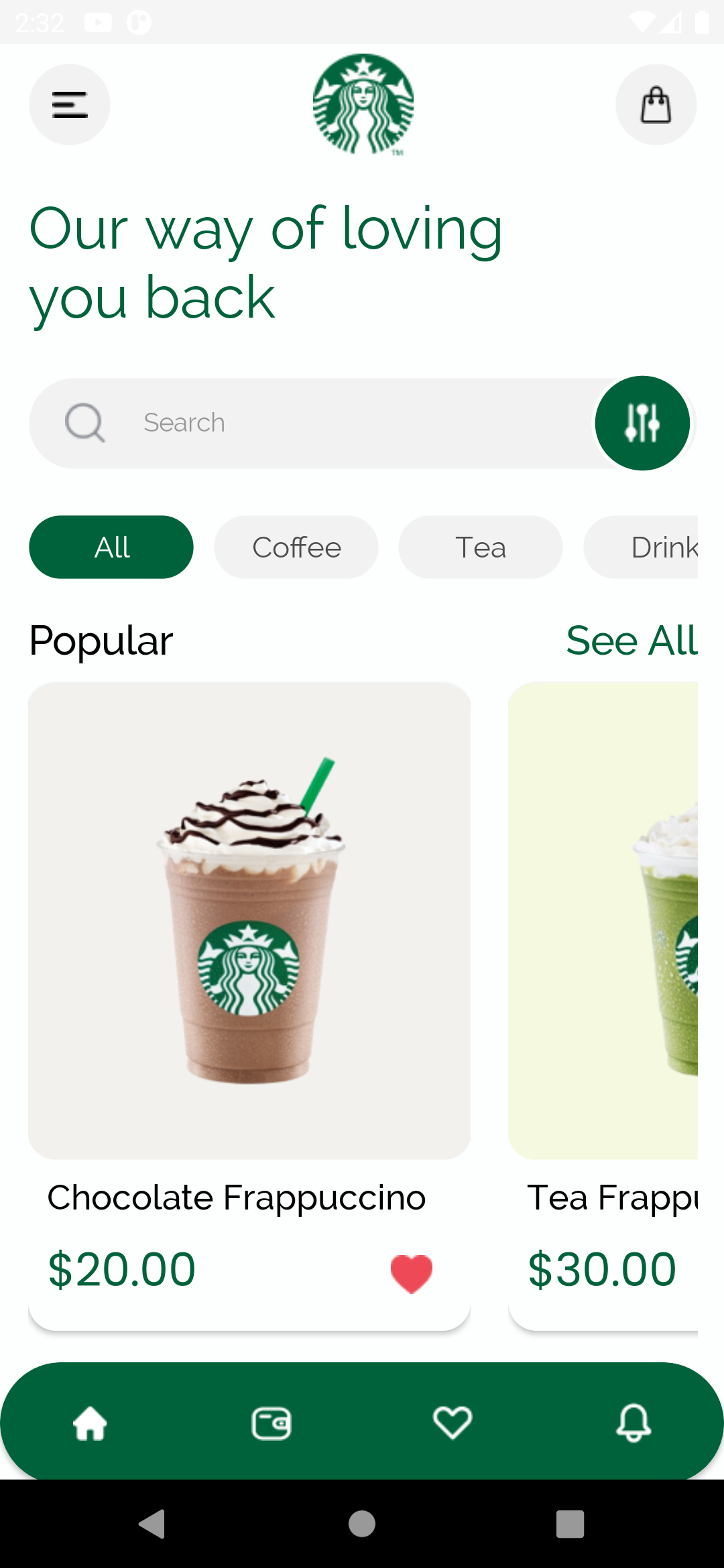The image showcases the Starbucks app on a smartphone screen. The background appears slightly blurred, but certain elements stand out distinctly. At the top, there is a strong Wi-Fi signal indicator and the recognizable Starbucks logo. The headline in green reads "Our Way of Loving You Back." Below the headline, there is a search bar. A list of purchasable items from Starbucks starts with the section titled "Popular." The first item displayed is an image of a Chocolate Frappuccino, priced at $20, which seems unusually high, suggesting the use of a different currency, possibly pesos. Next to it, there is a Tea Frappuccino priced at $30. 

At the bottom of the screen, the Starbucks app features a navigation panel with icons, including a house symbol for the home page, a card for adjusting your card balance, a heart for favorites, and a bell for notifications. Notably, the Chocolate Frappuccino has been favorited by the user, indicated by a heart icon. The phrase "Our Way of Loving You Back" might imply a special promotion or offer, though its exact meaning remains unclear.